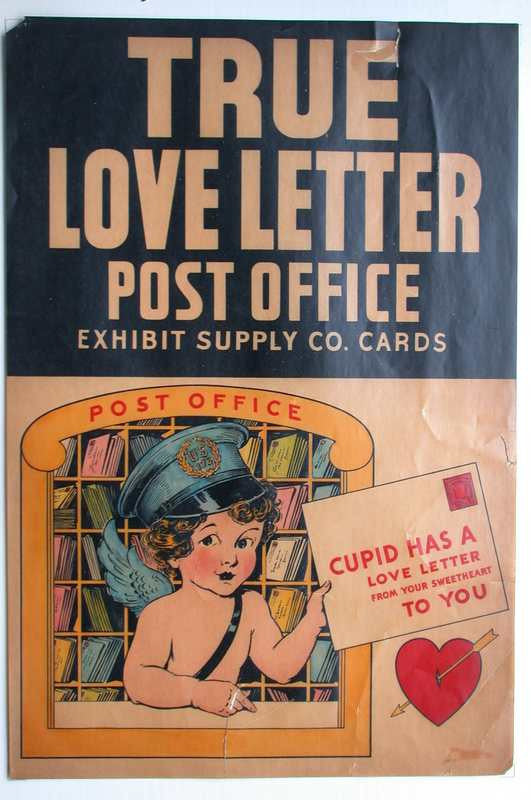This is an old-fashioned advertisement or poster, likely a scan of a small booklet or a piece of paper, featuring lively hand-drawn artwork. At the top, set against a navy blue background, bold white text reads, "True Love Letter Post Office Exhibit Supply Company Cards." Below this banner, the color shifts to an aged, slightly stained white background. At the center, a cherubic Cupid, identified by its small wings and wearing a blue and black postal carrier hat, sits at a little desk within a post office scene. Cupid is shirtless, with a strap running across its chest, and is depicted holding up a large letter inscribed, "Cupid has a love letter from your sweetheart to you." Surrounding Cupid are cubicle-like shelves filled with letters, and above the window where Cupid sits, "Post Office" is written in gold lettering. Attached to the letter Cupid holds is a red heart pierced by a yellowish arrow, adding a whimsical touch to this quaint and cartoonish design. The overall style is bright, featuring hues of blue, pink, and yellow, giving it a distinctly nostalgic and charming feel.